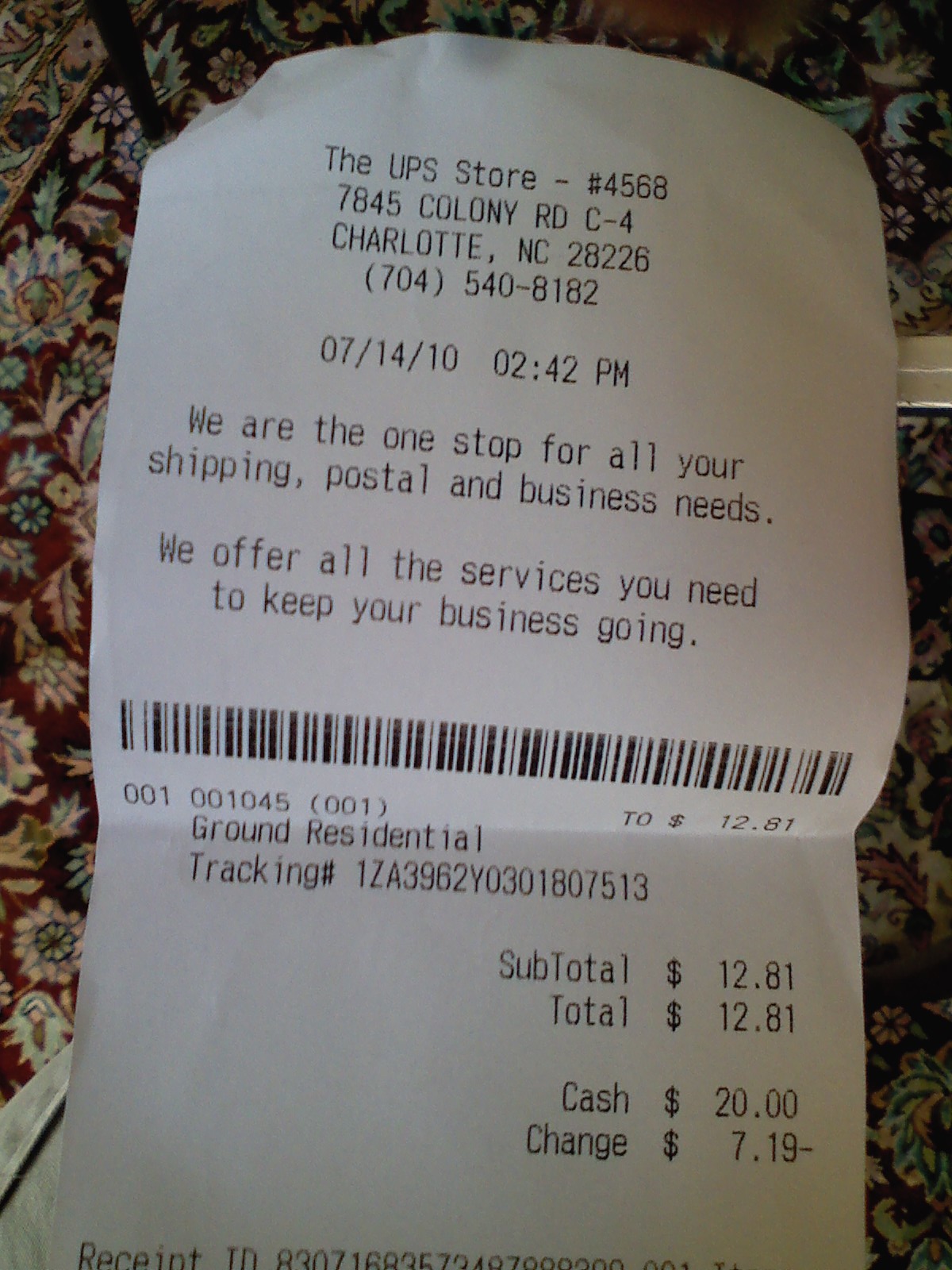The image displays a detailed receipt resting on a surface adorned with a flowery patterned material, which might be a tablecloth or possibly the arm of a sofa. The receipt is from the UPS store, specifically located at 7845 Colony Road, Charlotte, NC 28226, with the contact number 705-408-182x. Dated July 14, 2010, the transaction was made at 2:42 PM. The printed text on the receipt emphasizes that the UPS store is a comprehensive stop for all shipping, postal, and business requirements, offering a variety of services to support business operations. The cost for the delivery service was $12.81, paid in cash with a $20 bill, resulting in $7.19 as change.